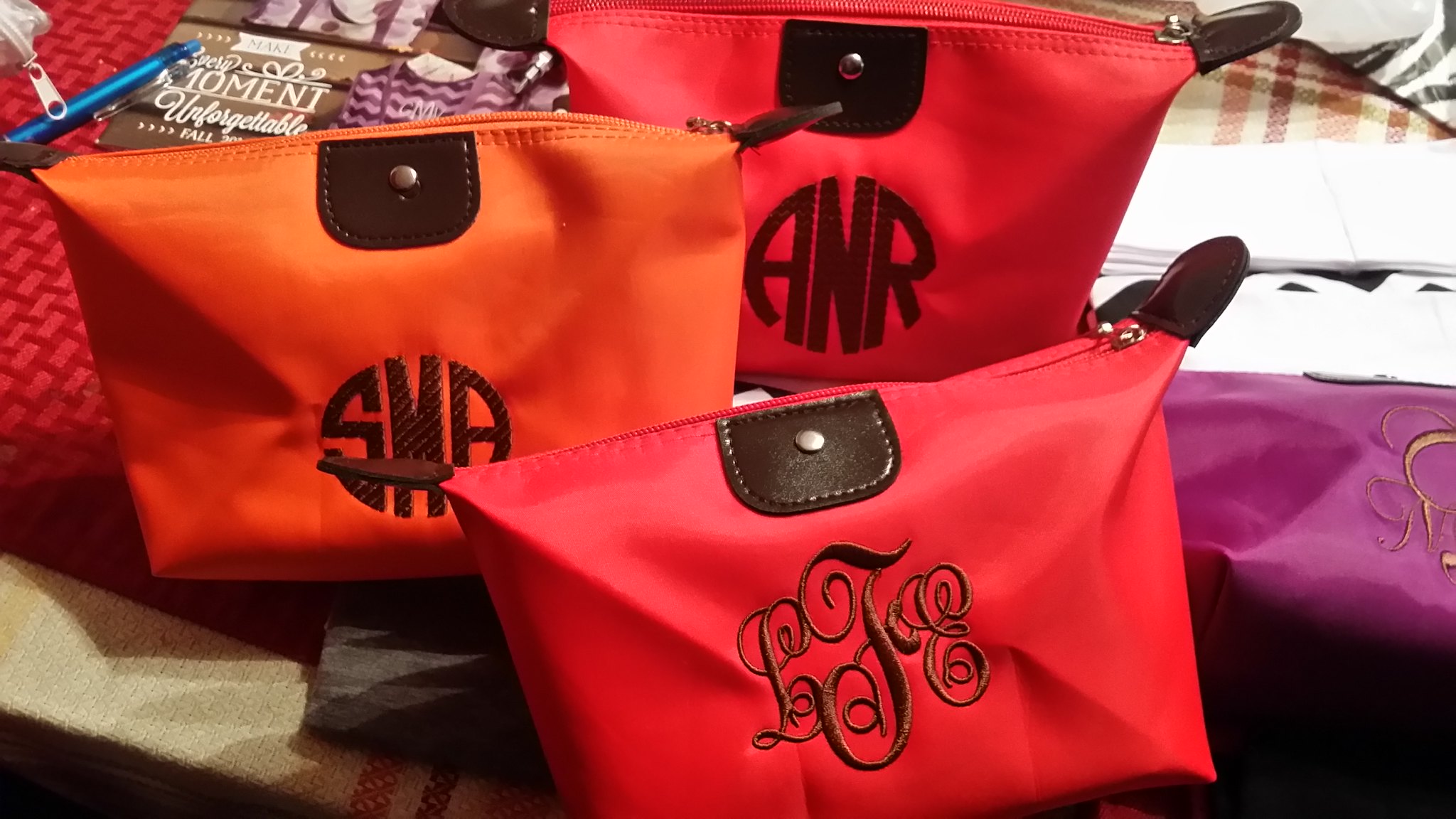In the image, we see four colorful cosmetic pouches displayed on a red bedspread with a rectangular pattern. The main focus is on three pouches arranged centrally. The pouch on the left is orange and features the initials "SMA" in block lettering, embroidered in brown with a brown leather tab and a silver zipper. Behind it, there's a red pouch with "ANR" initials, also in a circular pattern, distinguished by a black leather patch with a silver dot near the zipper. In front of these, slightly to the right, is another red pouch with "LTE" in elegant, swirly cursive, and a black leather area at the zipper. To the far right, a small portion of a purple pouch with an initial in brown is visible. The scene includes a blue pen, and a box labeled "moments, unforgettable" adds context, suggesting these pouches might be in a workspace where they are being stitched or engraved.